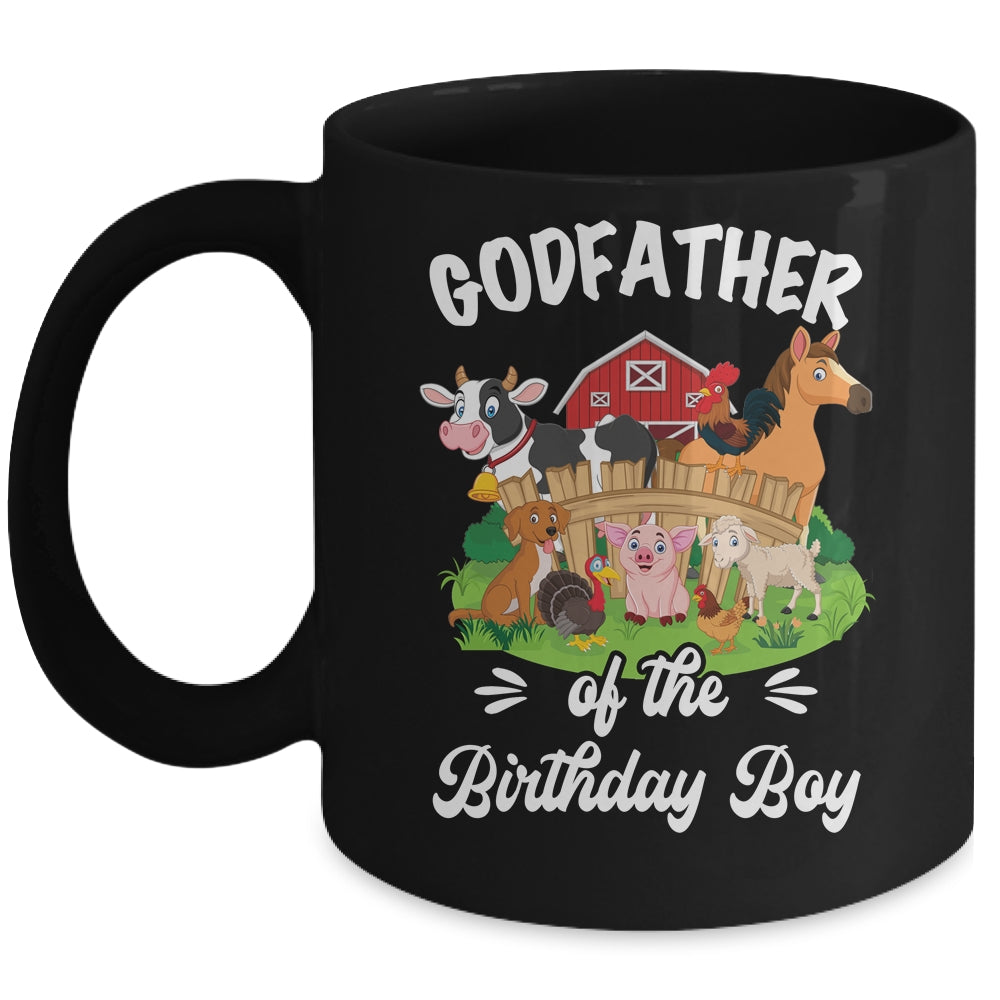This photograph depicts a charming black coffee mug with a vivid farmyard scene featuring various cartoon farm animals and a red barn, all set against a backdrop of green grass, flowers, bushes, and a brown fence. The mug bears white text that reads "Godfather of the Birthday Boy," with "Godfather" in bold letters at the top and "of the Birthday Boy" in cursive at the bottom. Centered between the text is a delightful illustration featuring a Holstein cow with a bell, a brown horse with a rooster perched on its back, a pink pig, a sheep, a turkey, a dog, and another rooster. This playful and detailed design makes the mug suitable for holding coffee, cocoa, tea, or any beverage, adding an extra touch of whimsy to any drink.